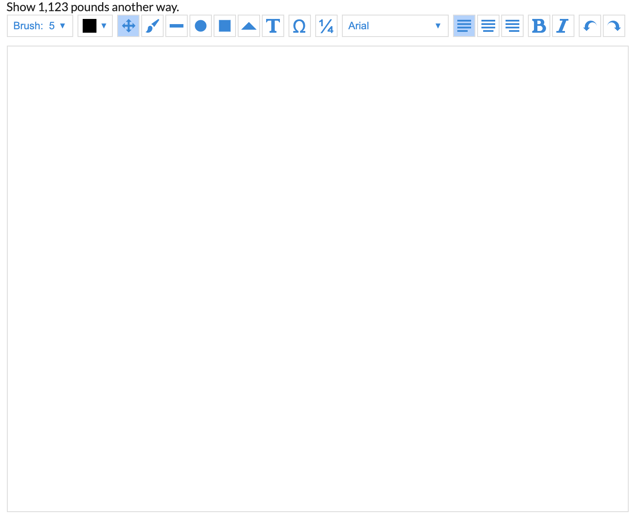The image depicts a screenshot of a text editing page, mostly blank with a light grey outline framing it. In the top left corner, there's some black writing on a white background, which reads "Show 1, 1, 2, 3, pounds another way." Below this text is a series of icons in a toolbar. The icons in the bar show a variety of tools: a brush with the number 5, a square, a smaller square with a cross inside, a paintbrush, a horizontal line, a circle, a square, a triangle, a "T" for text, an omega symbol, a quarter symbol, and various text formatting icons such as Arial font and alignment tools for left, centered, and right text. The left-aligned text icon is highlighted. There are also bold, underline, and possibly undo and redo icons. The overall impression suggests a text document interface, but the page remains blank apart from the described elements, and there seems to be a confusion regarding whether the phrase "1, 1, 2, 3, pounds" pertains to weight conversion (like from pounds to kilograms) or a financial value in British currency. The blank state of the document emphasizes the preparation for content that hasn't been entered yet.